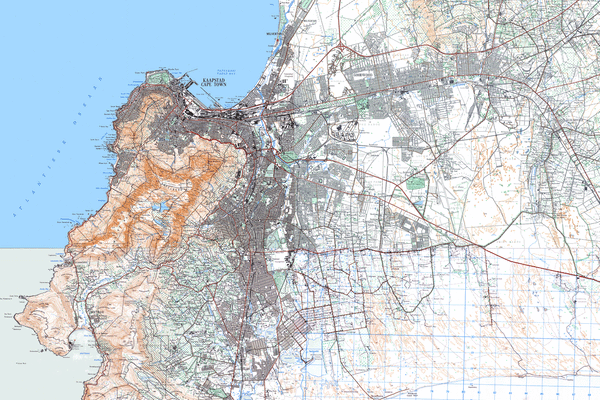The image depicts a detailed, digitally created map where gray and shades of orange dominate the color scheme, with areas of green, white, and minimal blue. The top left corner features a large, vibrant body of water labeled "Atlantic Ocean" and possibly "Cape Town," though the text is notably small and hard to read. The water region is encased in a darker, more colorful filter compared to the rest. The major portion of the land, which occupies the right side, is highlighted with various lines indicating roads and geographical segments, with colors including light blue, light orange, dark orange, light green, tan, and black. These colors shift in intensity towards the left, where the coastline with its vibrant contrasts stands out. The map appears to be less populated towards the right, encapsulating a specific geographical location with a semi-transparent white layer that mutes the vibrancy of the central and right areas.